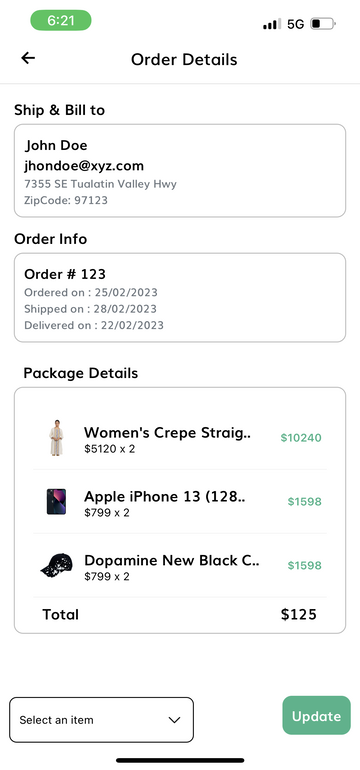Screenshot of cell phone display featuring order details: 

At the top, the time "6:21" is displayed in a light green button, accompanied by the cell phone reception icon indicating full bars, the "5G" network status, and the battery icon. Below the status icons, the image shows a header with a back arrow and the words "Order Details."

The first section, titled "Ship and Bill To," features the recipient's information:
- Name: John Doe
- Email: shayhondo@xyz.com
- Address: 7355 SE Tuleton Valley Highway, Zip Code: 97123

The next section, "Order Info," contains specific order details:
- Order Number: 123
- Order Date: Not specified
- Shipped Date: Not specified
- Delivered Date: Not specified

Finally, the "Package Details" section lists the items included in the order:
- Woman's Cap
- Straightener
- Apple iPhone
- Dopamine (New, Black)